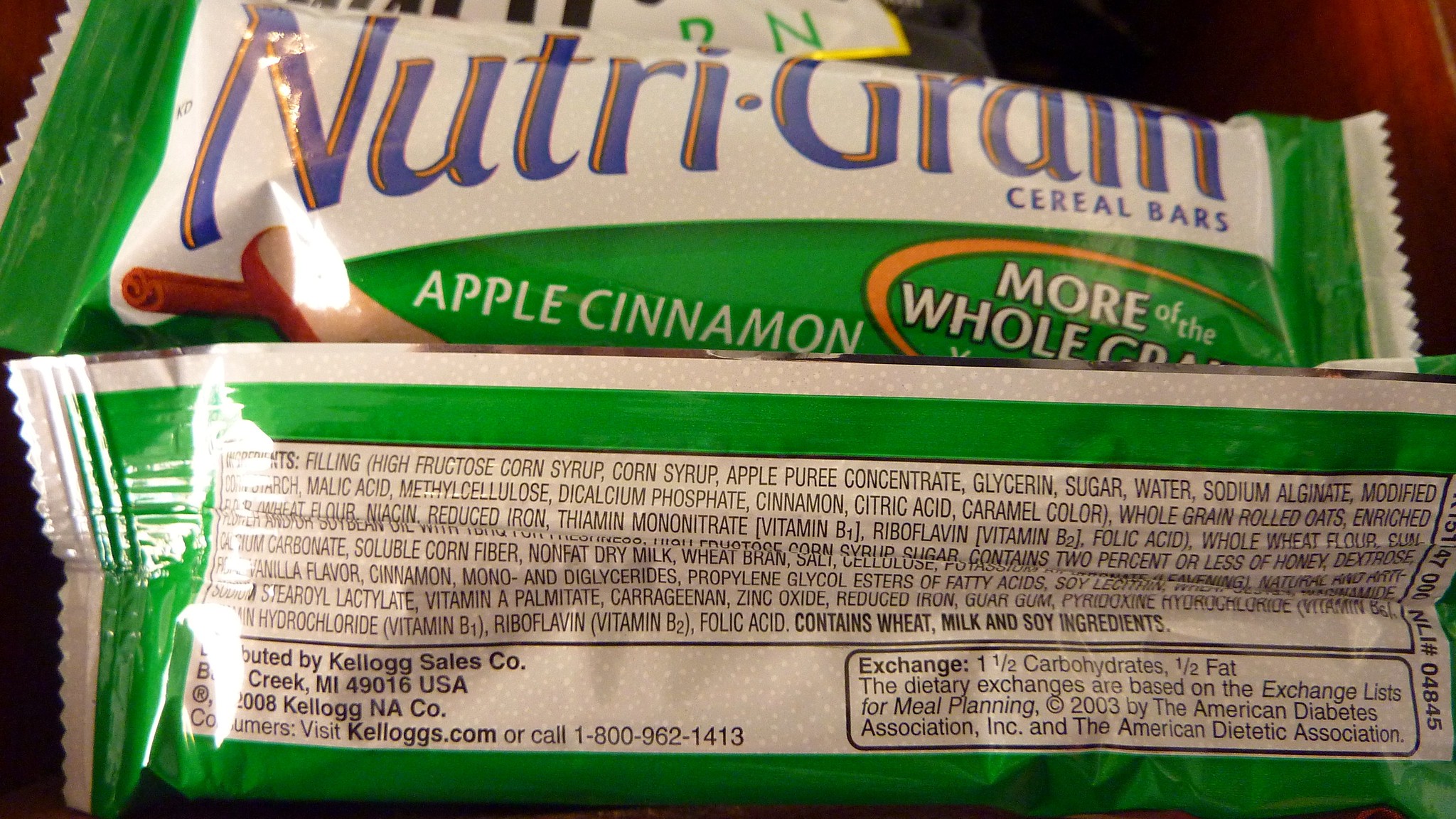A close-up image featuring a box of Nutri-Grain cereal bars set against a dark background. The box prominently displays "Nutri-Grain" in bold white and blue text at the top, while the bottom right corner clearly reads "Cereal Bars." Just below, the flavor "Apple Cinnamon" is indicated. To the right of the text, there's a round orange graphic, which likely promotes a specific nutritional benefit, though the exact wording isn't completely legible. The bottom section of the box is green and contains additional text, partially obscured by light reflections, that possibly details nutritional information or promotional messaging.